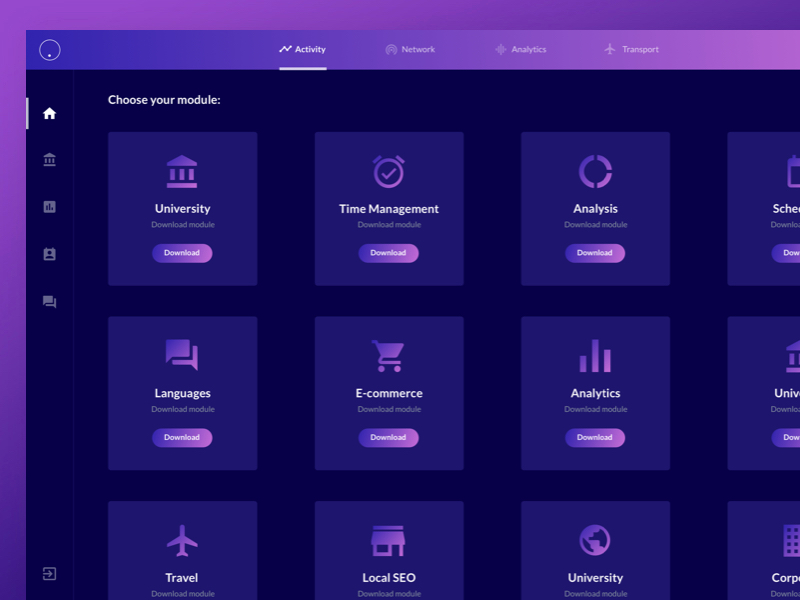This is a detailed screenshot of a website with a predominantly dark theme, featuring a combination of black, purple, and indigo hues, and white text. The main background of the site is a rich purple. At the top of the page, there is a gradient navigation bar that starts with an indigo shade on the left and transitions through various colors to mauve on the right. In the top-left corner of the screen, within this nav bar, there is a distinctive white circle that contains a smaller white dot at its bottom edge.

Central to this navigation bar are several menu options: "Activity," "Network," "Analytics," and "Transport." Directly beneath this is a black secondary navigation bar, also with a black background, which features the text "Choose Your Module" in white font.

On the left-hand side of the page, in the black section, there are several navigation buttons, each symbolized with different icons: a home symbol (currently highlighted to indicate the user is on the home menu), what appears to be a university building, an unidentified third symbol, a silhouette of a person, and a chat icon. At the very bottom of this left column is a square with an arrow pointing to the right, suggesting an option for more settings or actions.

The main part of the screen displays a grid of modules, each depicted as blocks arranged in four columns and three rows. The blocks are shaded in a navy or indigo color, with their logos illustrated in a mauve pink, and their names in white text. Each block also includes a "Download" button.

The modules are categorized as follows:
- The top row includes "University," "Time Management," "Analysis," and part of "Schedule" (which is partially off-screen).
- The second row lists "Languages," "E-commerce," "Analytics," and the beginning of another module starting with "UNIV" (the rest is obscured).
- The third and final visible row comprises "Travel," "Local SEO," another "University" module, and part of a module starting with "CORP" but not fully visible.

This caption provides a comprehensive description of the webpage's structure, design elements, and available navigation options.